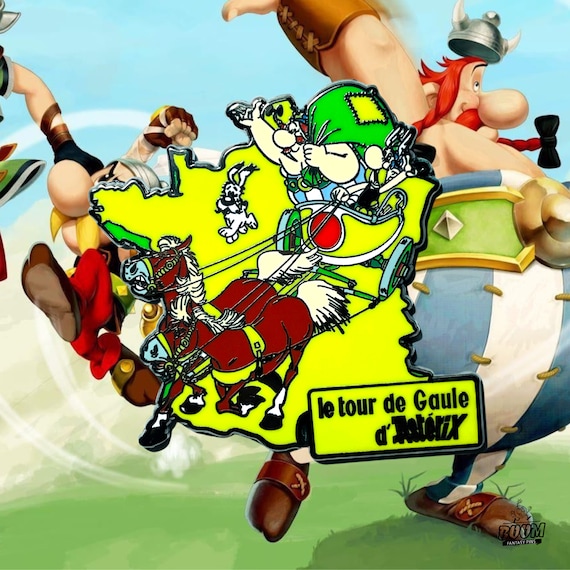This image is an advertisement for a game featuring a blend of illustration and 3D animation styles. Dominating the scene is a central cartoon graphic set against a vibrant yellow background. In this graphic, two brown horses pull a chariot ridden by a rotund, red-haired Viking character, who sports distinctive red braids, a red mustache, and a Viking helmet. He's depicted with a large green sack featuring yellow patchwork slung over his shoulder, reminiscent of Santa Claus. Accompanying him in the chariot is a small rabbit. Below this central illustration, the text "Le Tour de Gaulle" is prominently displayed, with some indiscernible text underneath. This centerpiece is surrounded by a 3D animated background where the same Viking character appears, equally large with a prominent nose, wearing white and blue pants, brown sandals, and a Viking helmet. To the side, partially obscured by the central graphic, stands another character with a yellow mustache. At the bottom of the image, the word "BOOM" draws attention with a small bomb figurine sitting above it.